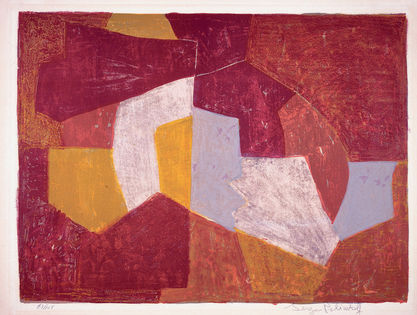This image depicts a modern abstract painting on a white piece of paper, filled with an amalgamation of vibrant colors and shapes. The painting prominently features different shades of red, occasionally interspersed with bursts of orange, light blue, and white. The various polygons and patterns appear to squish together, creating a dynamic and chaotic composition. Amid these interlocking shapes are white patches that introduce negative space into the artwork. The painting's title, "Composition Carmen, Brunet, Jaunet et Gris," reflects its rich color palette, which also includes maroon and gold. Created by Sergei Polyakov in 1956, this oil or pastel crayon piece has a landscape orientation and spans the full width of the paper while occupying about half the vertical space. Though the artist’s signature appears at the bottom of the piece, it is difficult to discern due to the zoomed-out perspective. The overall style is distinctly modern and contemporary.